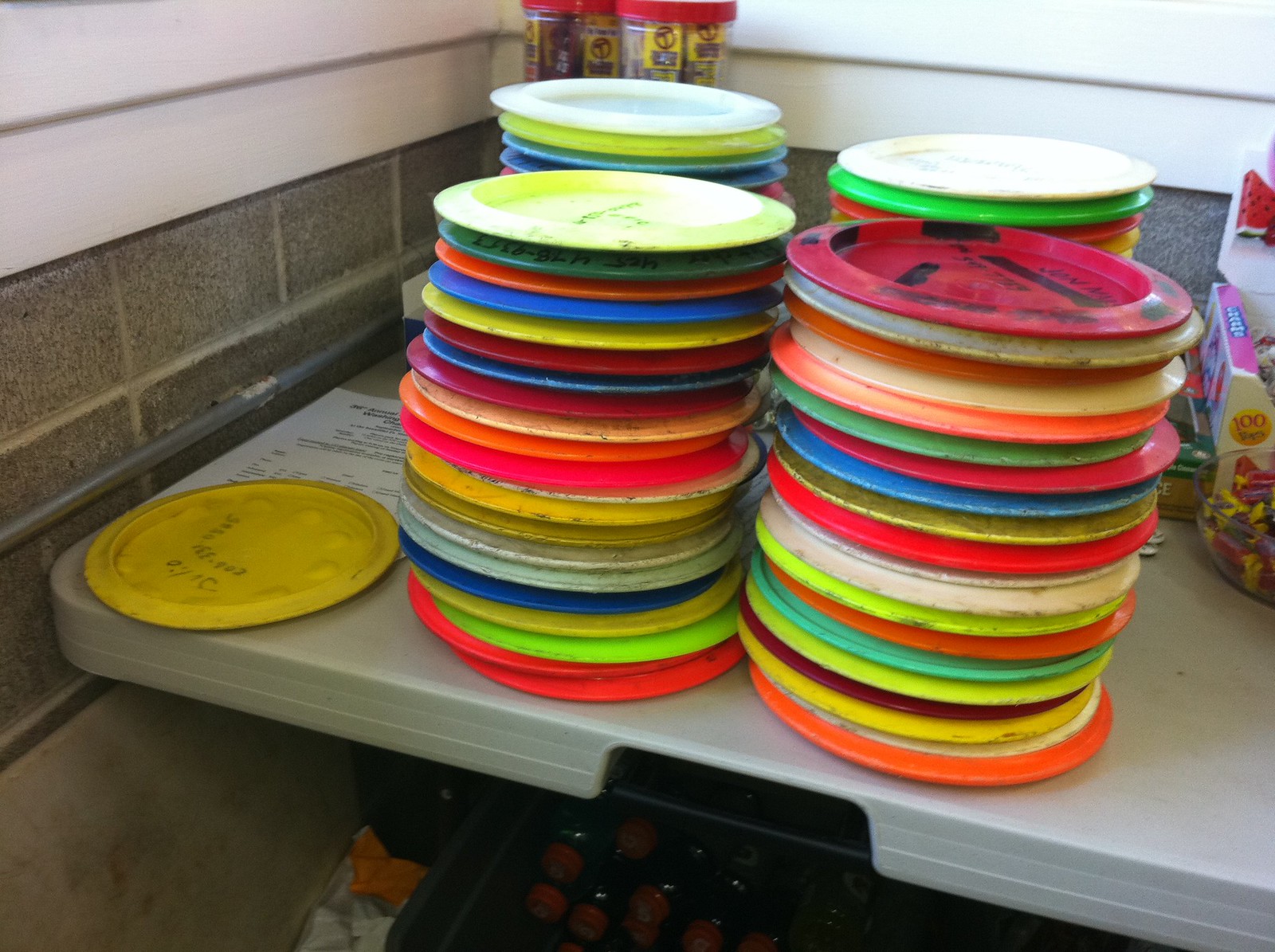The image captures a storage area within a school gym, showcasing a grey, portable plastic table commonly associated with camping or outdoor activities. On this table, there are four stacks of multicolored frisbees, arranged in two rows. Each stack contains approximately 17 to 18 frisbees of various colors, including red, orange, yellow, green, white, blue, pink, and mauve. The frisbees are visibly worn from use, with rough edges. To the left of these stacks sits a solitary yellow frisbee. 

In the backdrop, the walls feature a white finish with a dark brownish tile trim, converging at the corner where the table is positioned. The ground beneath the table remains obscured due to poor lighting. Additionally, to the right of the frisbee stacks, there are boxes and bowls containing assorted candies and two tubes with red lids, likely appealing to younger children. The scene's perspective is slightly to the right, emphasizing the colorful yet well-used frisbees as the focal point.